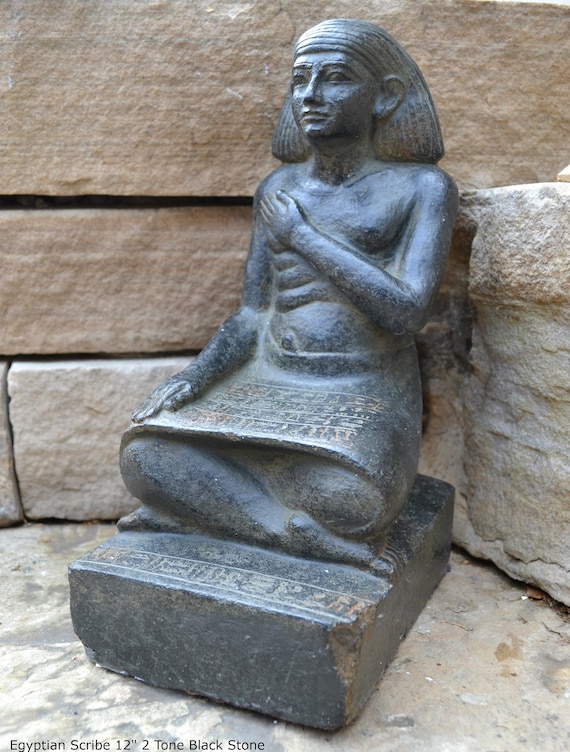The photograph depicts a detailed sculpture of an Egyptian scribe, carved from dark, charcoal-toned stone. The scribe is seated cross-legged on a black stone pedestal, which is adorned with rows of hieroglyphics along its front edge. His attire includes only a traditional Egyptian kilt that stretches over his legs, resembling a flat, tight surface, possibly indicated hieroglyphics as if he were holding a sheet. He is shirtless, and his left hand is positioned over the right side of his chest, while his right arm rests on his right leg.

The scribe wears a typical Egyptian headdress that drapes down the back, akin to those seen in Egyptian murals or on pharaoh statues, with his ears and facial features distinctly visible. The pedestal and the statue share the same dark, almost black color, creating a unified and somber aesthetic. The statue is set against a backdrop of large, light-brown, tan blocks, which form the corner of the two walls behind it. The ground in the photograph appears to be a white stone surface, contrasting sharply with the dark sculpture. The bright daylight illumination in the image allows for a clear view of the detailed craftsmanship and texture of the statue and its surroundings.